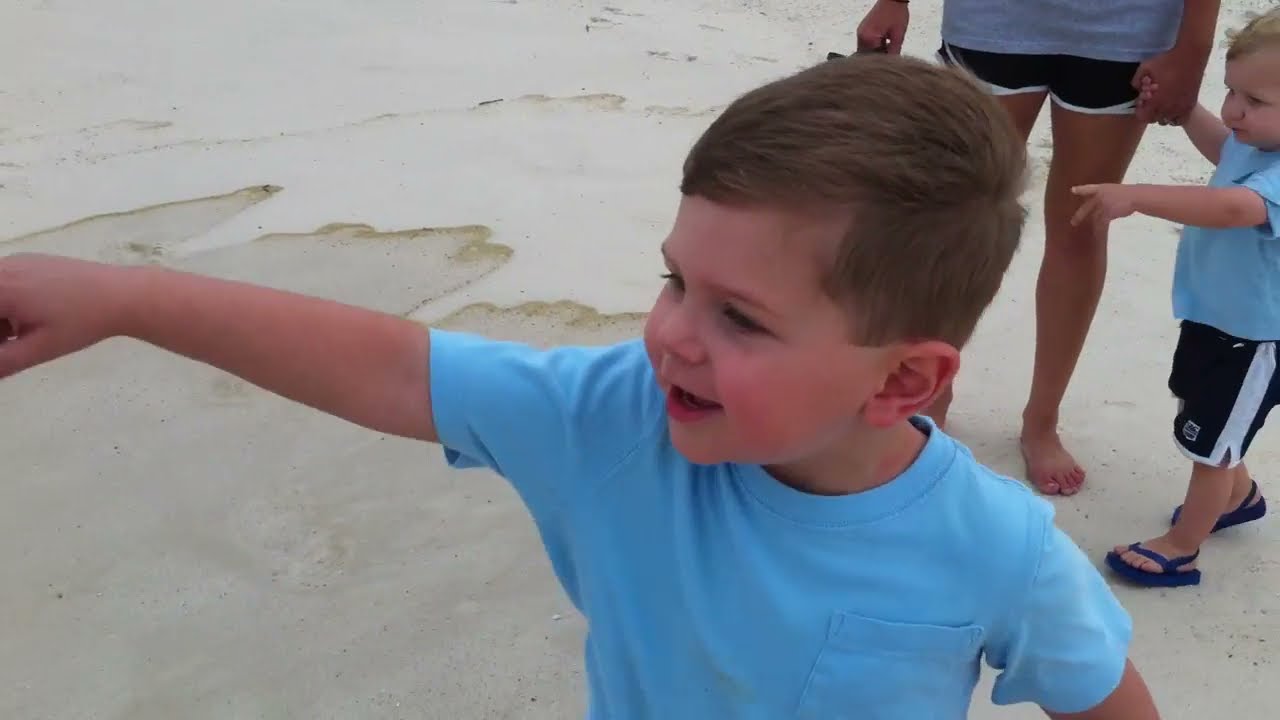In this image set against the backdrop of a pockmarked sandy beach with small pools of water, there are two young boys and an adult who appears to be their father. The two boys, both with light brown hair and dressed identically in light blue t-shirts and blue shorts with white stripes down the sides, are visible. The older boy, in the foreground, is around 5 years old and is pointing enthusiastically towards the ocean. His face radiates excitement and delight as he gestures with his arm extended. The younger boy, appearing to be around 2 or 3 years old, is holding the hand of the father, who is partly visible from the waist down, also dressed in a matching light blue t-shirt and blue shorts. The father's right hand is clenched around an unseen object. Both boys are seemingly captivated by something in the direction they are pointing, sharing a moment of curiosity and wonder. The family appears connected and content, enjoying their time together on the beach.